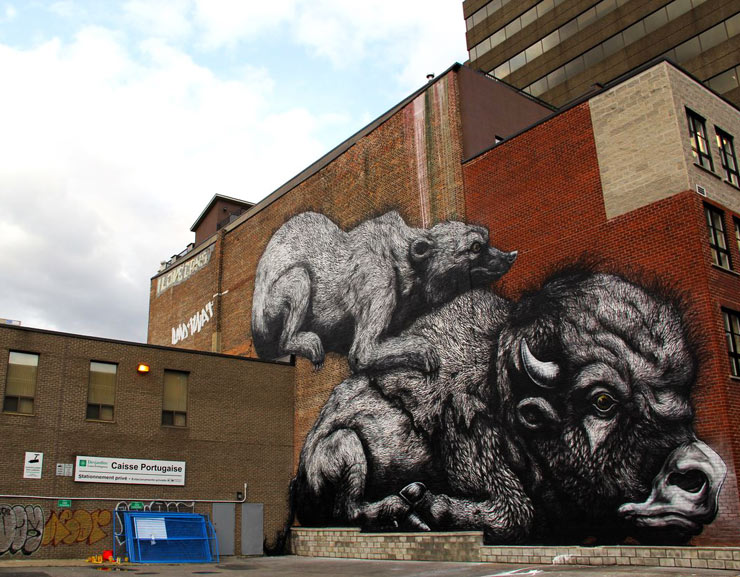In this image, we are observing the exterior of a building adorned with a detailed mural. The mural features a powerful gray and black bull with prominent white horns. Perched on the bull’s back is a light gray animal, resembling a hyena, depicted in a side view. 

At the bottom of the image, there is a light gray ground base. In front of this base stands a small brick-styled wall, composed of four rows of bricks, with an extension of just two rows to the right. Adjacent to this setup is a small brown building, which displays a white rectangular sign. This sign is marked by graffiti art in shades of gray and orange. Beside this building on the right are blue fences.

The much taller building is painted reddish-brown on the front and brown on the back. To the top right of the mural, another skyscraper is visible, characterized by its brown and gray facade. The left-hand side of the image reveals a predominantly white sky.